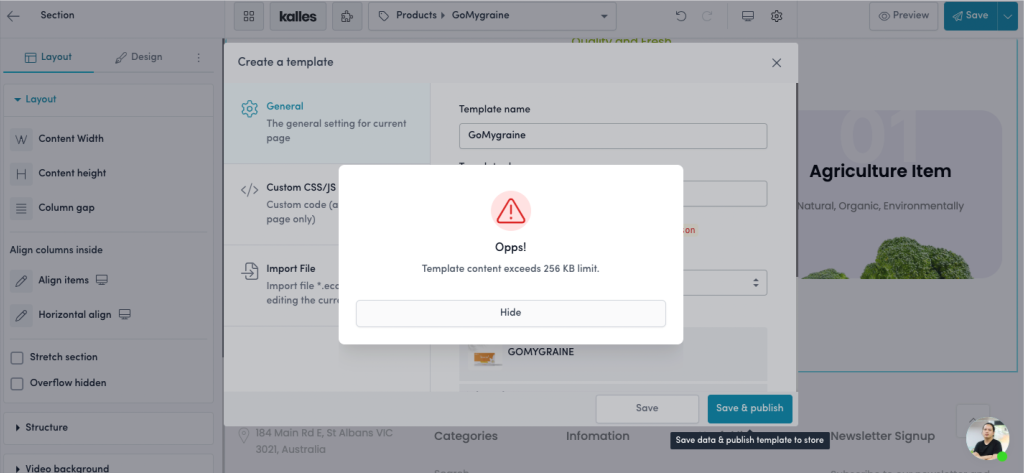The screenshot depicts a user's desktop, featuring a central pop-up window prominently displayed against a backdrop of a web page and another semi-translucent pop-up window. The central pop-up is white, adorned with a red exclamation point inside a triangle and a pink circle. Below this, a message reads: "O.P.P.S. Template content exceeds 256 KB limit." A "Hide" button is presented below the notification.

Further down, the page transitions into a "Create a Template" interface with sections labeled "General Settings," "Custom," and "Import File." Various scroll-down menus and input boxes populate this area, accompanied by "Save" and "Save & Publish" buttons. The underlying web page, slightly obscured by the pop-ups, includes a vertical scroll bar on the left and a horizontal header with the text "K.A.L.L.O.S."

Adjacent to the header, there's a dropdown menu labeled "Products," along with "Preview" and "Save" buttons. One visible item within the pop-up to the right is described as "Agriculture item, natural, organic, environmentally," next to an image resembling broccoli. In the lower right corner of the screen, a small circular profile picture with a tiny green dot is visible, indicating the user’s online status.